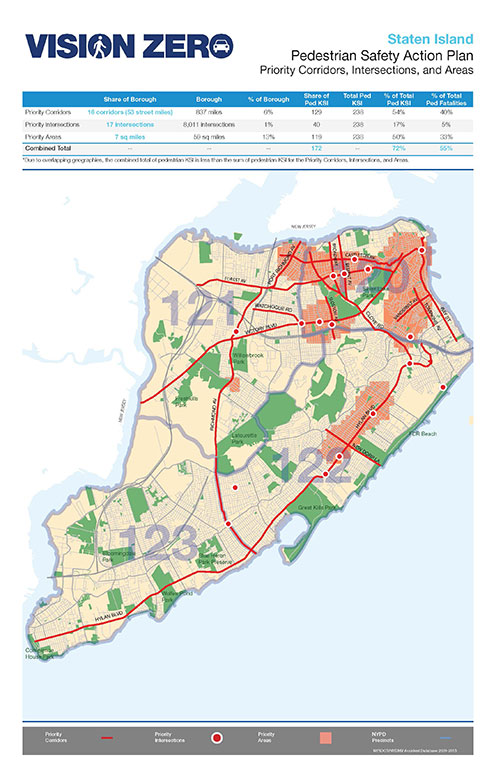This color poster, featuring Staten Island's Pedestrian Safety Action Plan, prominently presents a detailed map at its center. At the top left, bold text spells out "Vision Zero," with integrated white images of a stick figure pedestrian and a vehicle within the letters. On the upper right, light blue text labels the area as Staten Island, followed by black text that reads, "Pedestrian Safety Action Plan: Priority Corridors, Intersections, and Areas."

The map itself highlights various details: light brown land sections, green areas indicating grassy regions, and red sections alongside certain highlighted roads. Numbers such as 120, 121, 122, and 123 mark specific points. The map is bordered by light gray, with blue water surrounding it and New Jersey in white to the left.

Below the map, a guide displays details in a combination of black, white, and blue text. At the bottom, a gray band contains detailed white text and an index to the map’s referenced elements. Additional writings, including possibly an NYPD designation, are present but not fully legible. Overall, the poster effectively communicates priority safety areas and evacuation routes for Staten Island pedestrians.